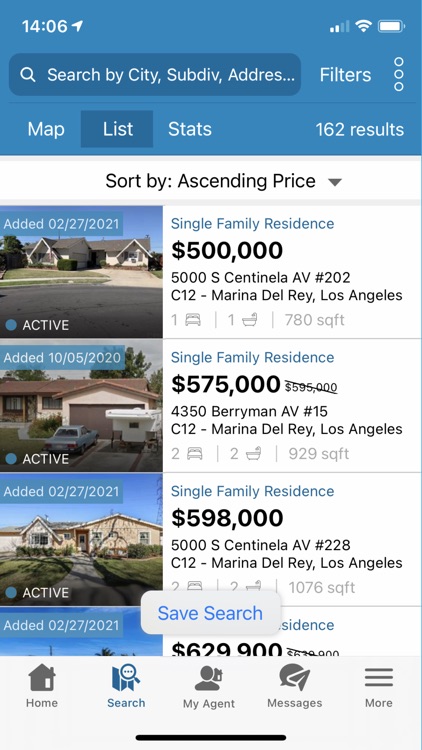This image depicts a real estate application interface. At the top, a blue banner displays "1406" alongside an Upward logo. The status bar includes icons indicating a full Wi-Fi signal and a fully charged battery, both arranged horizontally.

Below the banner, there's a search bar labeled "Search by city, subdivision, or address," accompanied by filter options and three vertically-aligned dots. Just beneath, a section with tabs labeled "Map," "List," and "Stats" shows "List" highlighted, indicating that the list view is currently active. This section also states "162 results."

Underneath, users can sort the listings by price in ascending order, indicated by a gray downward arrow. The main content area features images and details of three homes:

1. **5000 South Centinella Avenue, #202, Marina Del Rey, Los Angeles**
   - Type: Single-family residence
   - Added: 02-27-2001
   - Features: Driveway, sidewalk, front lawn with green grass, angled roofline on both sides.

2. **4350 Barry Mann Avenue, #15, Marina Del Rey, Los Angeles**
   - Price: $575 (reduced from $595)
   - Type: Single-family residence, single-story
   - Added: 10-05-2020
   - Features: Brown roof, brown two-car garage, trailer similar to a vacation camper on the right, blue sedan on the left of the driveway, left-hand walkway, two visible windows.

3. **5000 South Sentinel Avenue, #228, Marina Del Rey, Los Angeles**
   - Type: Single-family residence, single-story
   - Features: Beige exterior, front paved walkway with grassy areas on both sides, pitched roof on the left side.